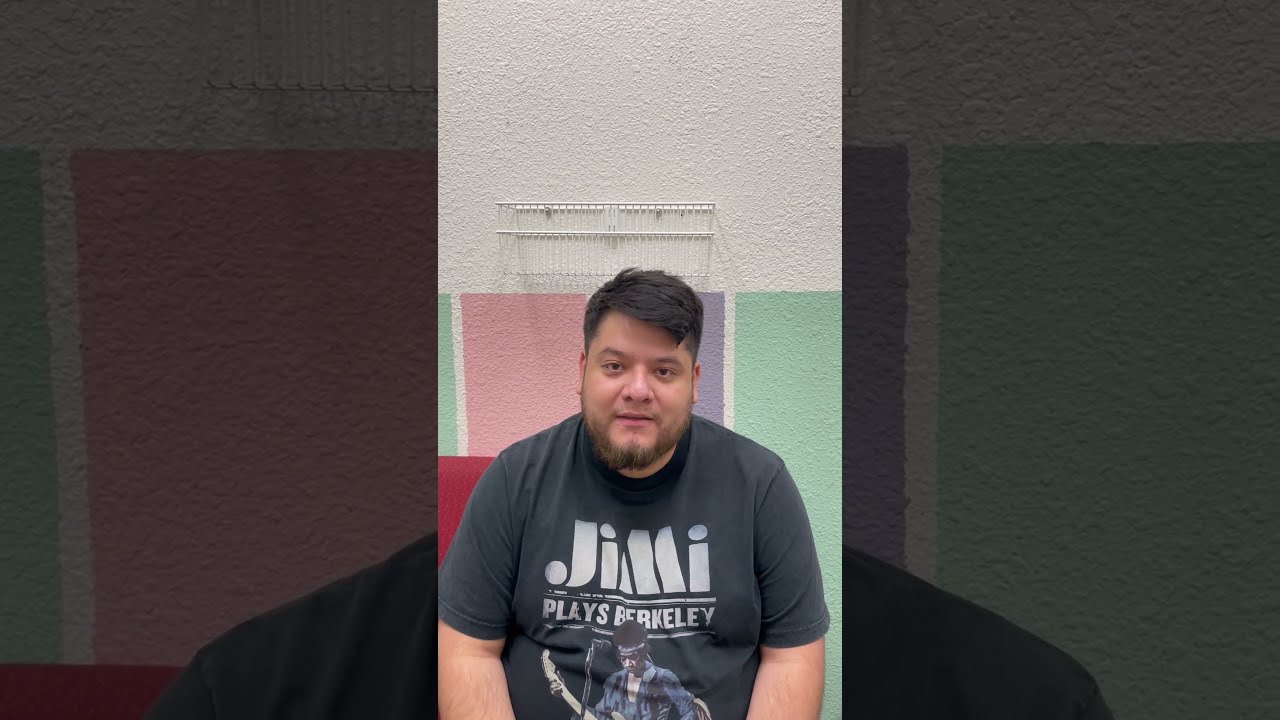In the center of the image, a man is sitting at the edge of a red chair, his posture relaxed against a colorful, geometric backdrop. Likely in his late 20s or early 30s, he sports short black hair with a thicker top and trimmed sides. His facial hair is denser on the chin, tapering up to lighter sides without a mustache, forming a neat goatee. He wears a black short-sleeve t-shirt featuring a graphic of Jimi Hendrix with a headband and blue jean jacket, playing a guitar next to a microphone. The text on the shirt is bold, with "JIMI" in capital letters and "plays Berkeley" underneath. Behind him, the wall is adorned with visually striking green, pink, and purple rectangles below a white section, adding a vibrant contrast to the scene. Flanking this central image are two zoomed-in, darkened fragments of the same picture, focusing on different aspects of the man and his surroundings, which include a vacant rack on the wall.